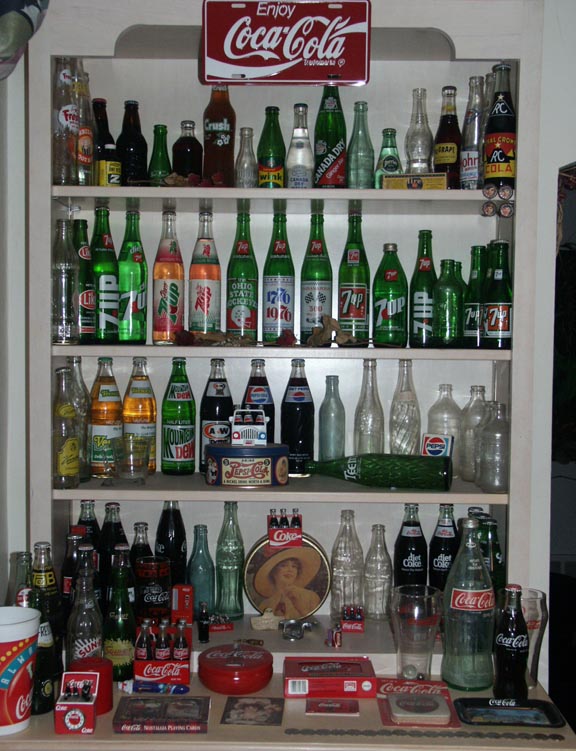The image depicts a white four-level shelf completely filled with an array of older-looking soda bottles, some still full and others empty. At the very top of the shelf, an attached red and white sign resembles a car license plate and bears the inscription "Enjoy Coca-Cola." The top shelf is densely packed with various bottles, including recognizable ones such as Crush. Descending to the second level, the majority of the bottles are vintage 7-Up. The third level showcases a mix of Mountain Dew, A&W, and Pepsi bottles. The bottom shelf, and the area directly in front of it, predominantly features Coca-Cola products. In addition to the bottles, the base of the shelf displays a miscellany of Coca-Cola memorabilia, including a cup, a book, some coasters, and a bunch of coins that might fit the Coca-Cola theme. Also present is a round photograph of a girl with a large straw hat, posed with her hands under her chin and smiling. She adds a nostalgic touch to this compelling collection.